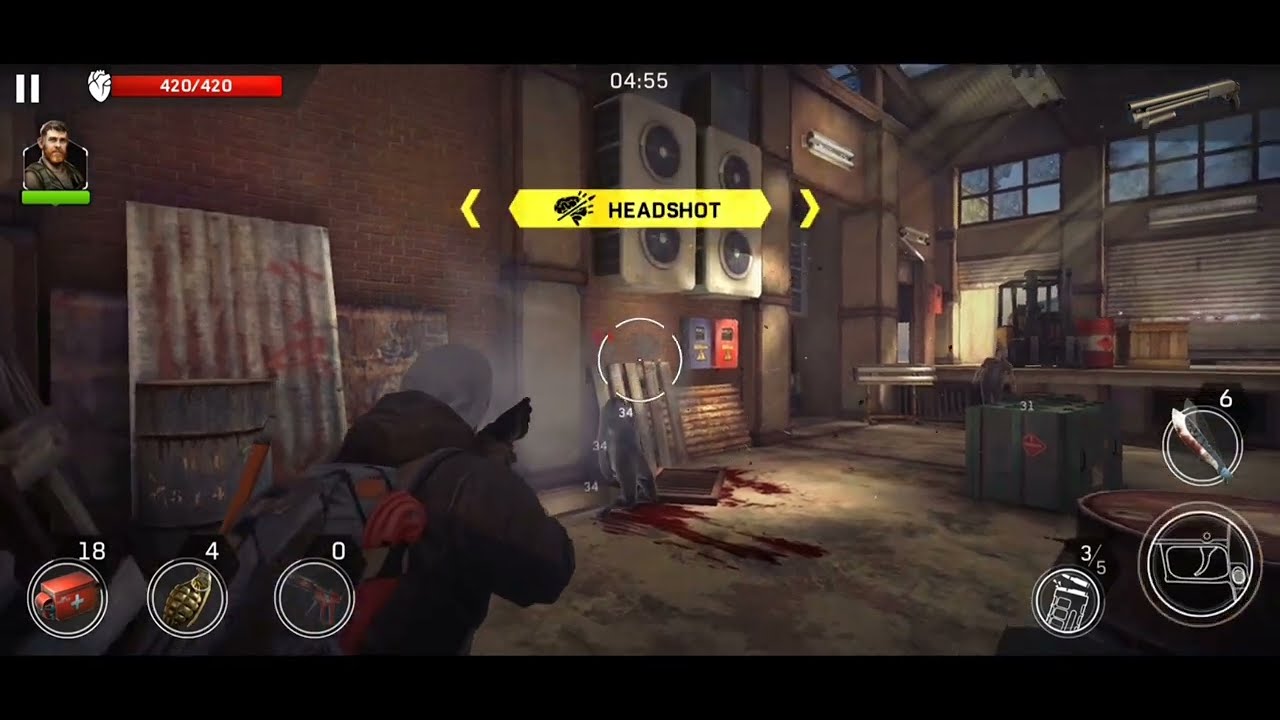This image is a detailed screenshot of a shoot-em-up video game set inside a dilapidated warehouse. The central figure in the screenshot is the main character, a Caucasian male with a brown beard and mustache, who is dressed in a layered outfit: a white hoodie underneath a green jacket, with a gray and orange backpack. He is pointing a rifle forward, ready to shoot.

In the top left corner of the screen, the player's status is displayed, including a health bar and numerical indicators showing "424/420," with an image of a white heart and a red bar. Beside this, there is a smaller image of the character’s head and shoulders. The center top of the screen shows the time as "04:55" along with a yellow banner featuring a brain pierced by a bullet, signaling a "headshot." Beneath this banner, the lifeless body of an enemy character lies headless, with blood splattered on the floor and wall, emphasizing the violent nature of the game.

In the lower left corner, three circular icons depict the player's available resources: the first circle shows an ambulance icon next to the number "18," indicating health packs; the second shows grenades and the number "4"; and the third circle is blurry, but faintly reveals a landmine icon with the number "0" beside it. The right-hand side of the screen displays the gun's trigger and barrel, while centrally, a round target area can be seen for aiming and shooting.

The environment is a rundown warehouse, with business features such as air conditioning units mounted on brown walls, and a benchtop visible to the right. Overall, the game's color palette primarily consists of browns and grays, contributing to the gritty, abandoned atmosphere.